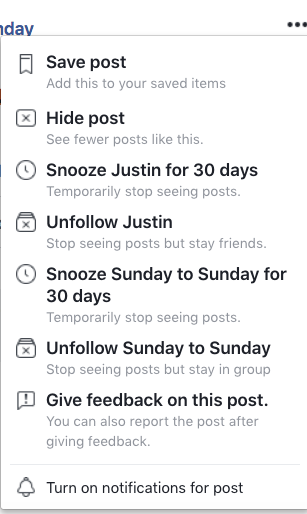This image captures a screenshot from a mobile phone, displaying a social media interface with various post interaction options. At the top of the screenshot, there's a bookmark icon next to the text "Save Post," along with a description below it saying "Add this to your saved items." Following that, there’s an option labeled "Hide Post" featuring a box with an X inside. Next, there's an option to "See fewer posts like this" that users can click on. Below that, a clock icon accompanies the text "Snooze Justin for 30 days," indicating the ability to temporarily stop seeing posts from a user named Justin. The next option, "Unfollow Justin," marked by an X in a box, allows users to stop seeing posts from Justin while still remaining friends. The interface continues with an option to "Snooze Sunday to Sunday for 30 days," again enabling the temporary hiding of posts. Farther down, there's another "Unfollow Sunday to Sunday" option with an X in a box. At the bottom of the screenshot, there’s a prompt to "Give feedback on this post," inviting users to provide input on the content they are viewing.